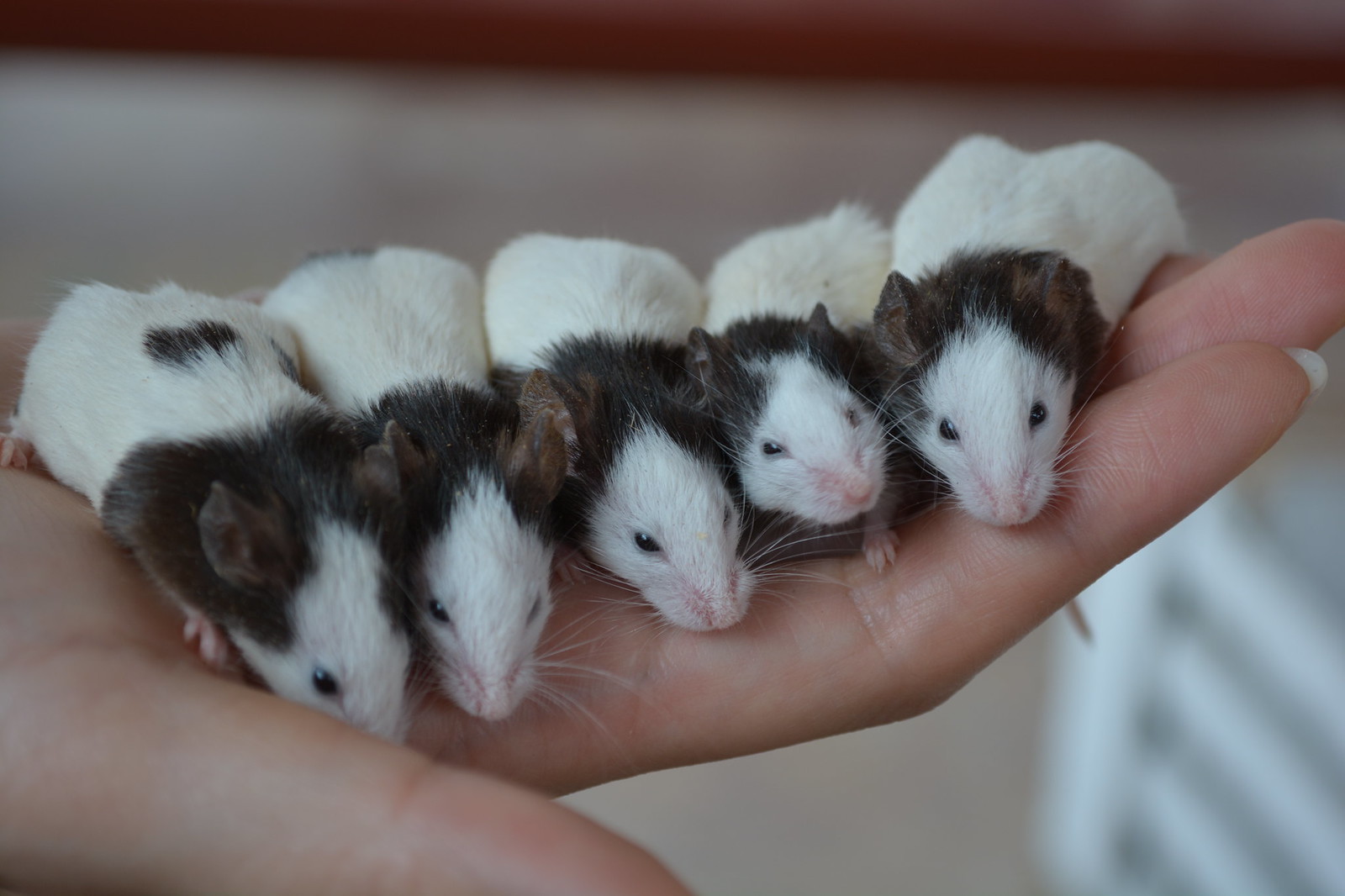In this image, a Caucasian hand with long fingernails—particularly a long white-tipped nail on the index finger—cradles five baby mice in its palm. The tiny mice, small enough to fit comfortably in the person's hand, exhibit a striking contrast in coloration: they are predominantly white with black fur encircling their necks and covering the tops of their heads. Each mouse has small, black beady eyes, white whiskers, and delicate pink ears and noses. One can pinpoint minor variations among them, such as a black patch on the back of the mouse on the far left. Their tails are mostly hidden, except for one faintly visible and blurred tail hanging over the fingers on the right. The background of the image is blurred with indistinct white elements, placing focus on the tender scene of these tiny creatures huddled together and gazing towards the camera.